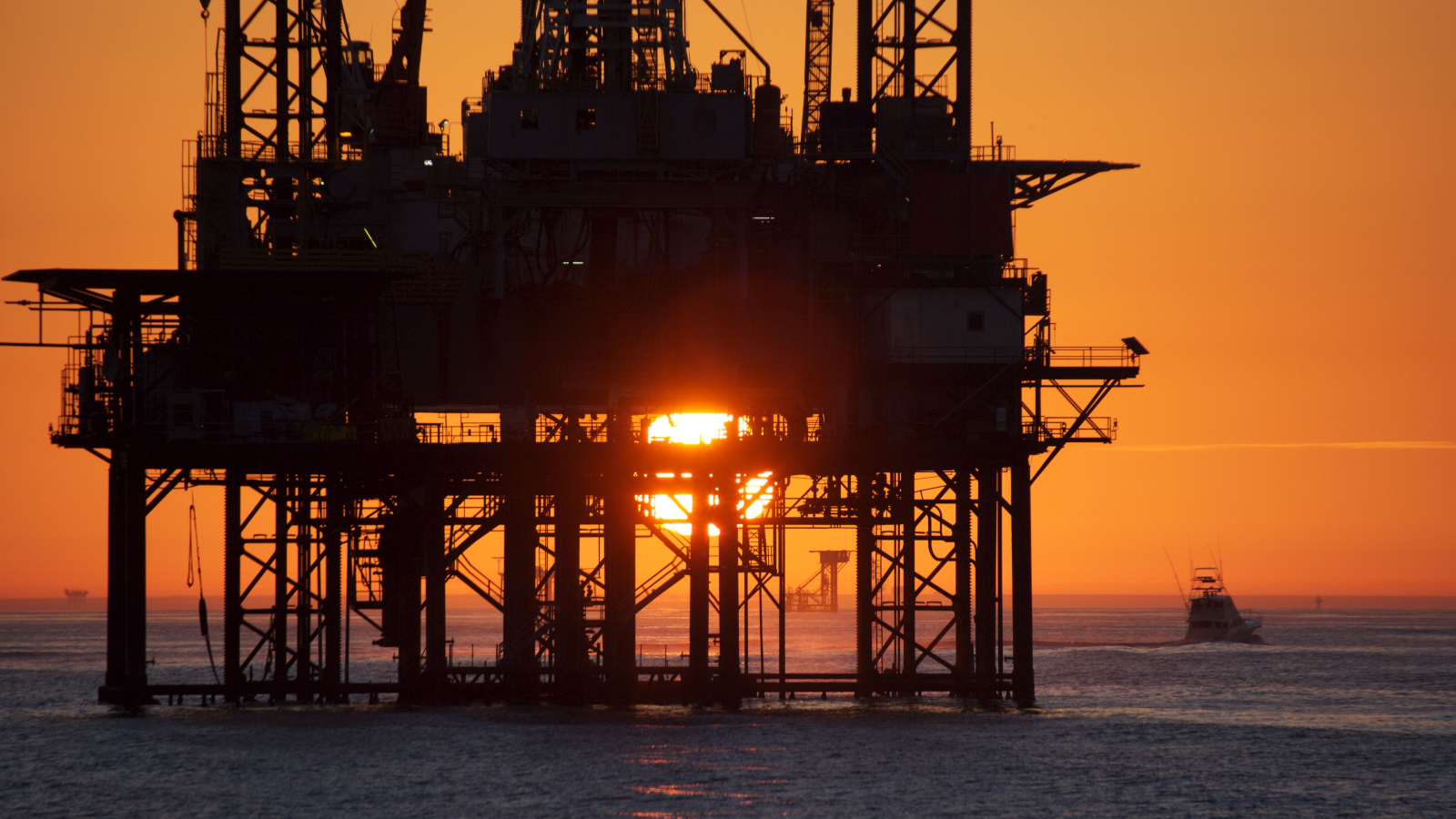A stunning photograph captures an oil rig silhouetted against the vibrant colors of a setting sun, positioned to the right of the image. The sky is ablaze with beautiful shades of orange and pink, casting a warm glow over the scene. Silhouetted against this backdrop, the dark outline of the oil rig rises dramatically, with tall stacks extending upwards—so tall that the top is cut off by the frame. The rig's base is obscured by the tranquil grayish-blue water, which stretches out to the horizon. To the left of the oil rig, a similarly silhouetted boat can be seen on the water's surface. The serene, reflective waters envelop the scene, accentuating the dramatic interplay of light and shadow created by the setting sun. This exquisite image, with its rich details and vivid colors, offers a serene yet powerful depiction of industrial silhouettes against a natural masterpiece.